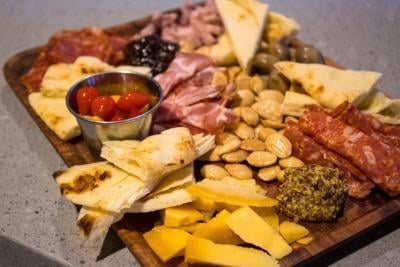The image depicts an enticing charcuterie board set against a gray background. The long, dark-stained wooden board is richly adorned with an assortment of delectable foods, showcasing a variety of meats, cheeses, and accompaniments. At the top of the board, a small, metallic ramekin likely filled with cherry tomatoes or olives sits as a focal point. Surrounding it, there are pita bread slices and a hardened dark yellow cheese positioned nearby. Scattered across the board, you can find various meats, including salami slices in the lower right section, and other meat variations throughout the middle and top parts. The lower section also features different types of cheese, interspersed with olives, completing this visually appealing and appetizing spread. Despite the somewhat haphazard arrangement, the board offers a delightful array of snacks perfect for grazing.